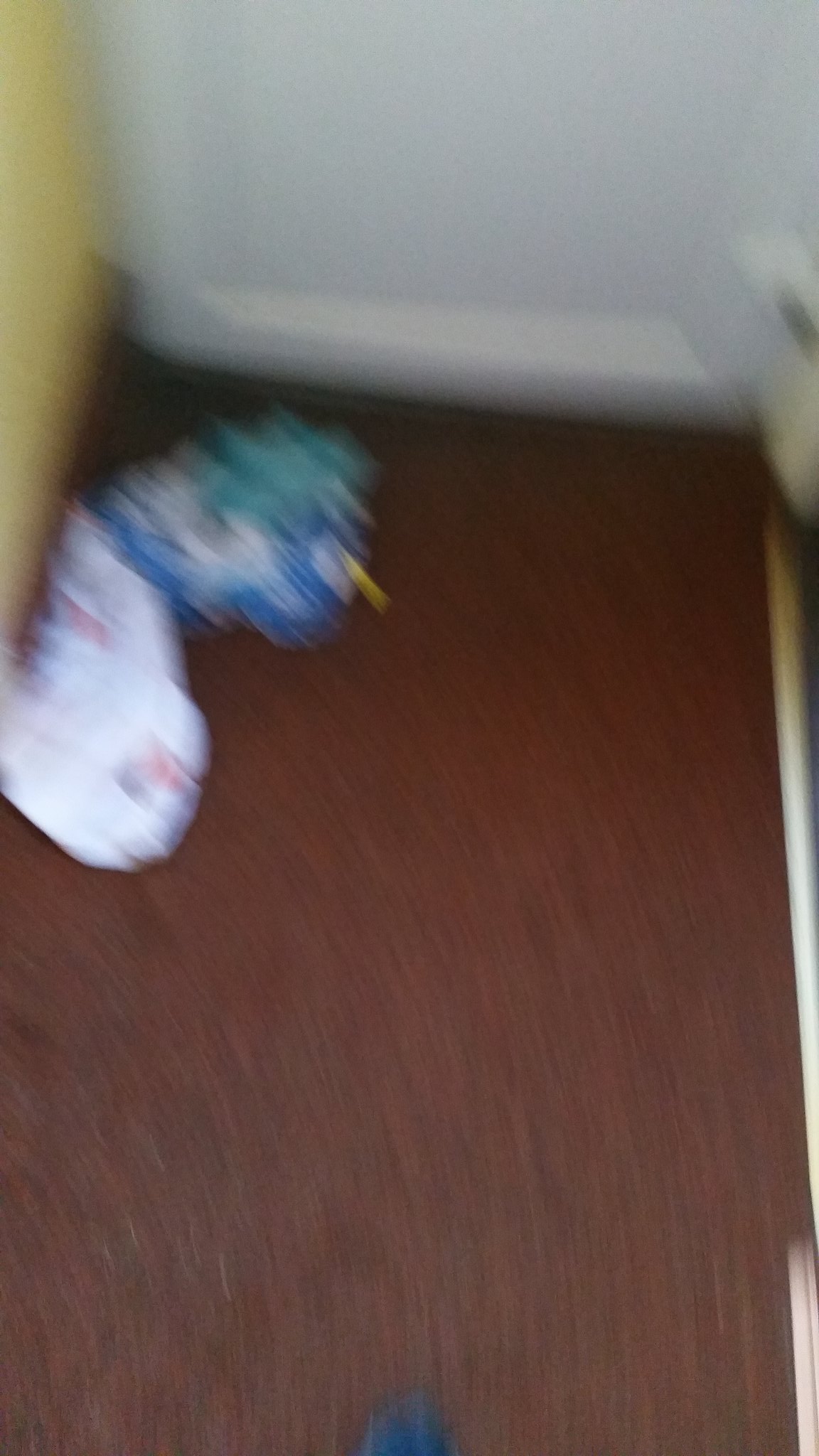A blurred, vertical portrait-oriented photograph captures the interior of a house. The floor, a distinct reddish-brown hue, is scattered with indeterminate items, featuring shades of white and green, possibly toys. The background showcases a white door framed by yellow walls, though the out-of-focus nature of the image renders other details indistinguishable.